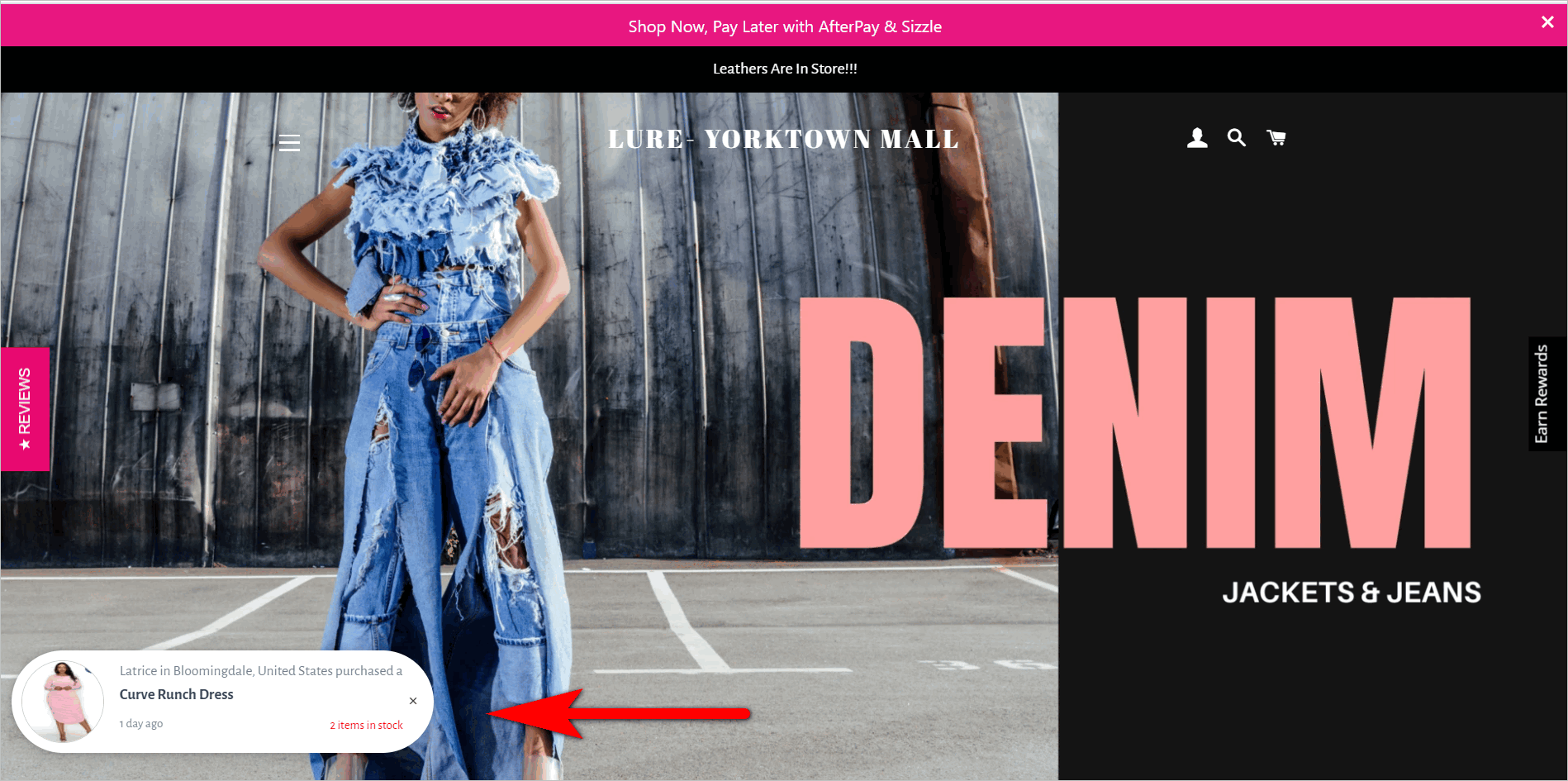A fashion website, potentially named "Lower Yorktown Mall," showcases trendy clothing with a stylish, inviting theme. The website prominently features a "Shop Now, Pay Later" option with Afterpay or Sezzle at the top. Emphasizing its focus on denim, the site has the word "DENIM" displayed in large, light pink letters, creating a striking contrast against the black and pink background colors.

One of the main images features a model wearing a distressed denim jacket and jeans, highlighting the quality and aesthetic of their denim collection. In the bottom left corner, there is an image of a curvy ranch dress, suggesting that the store offers both plus size and regular size clothing. The overall design and presentation of the website are visually appealing and designed to attract customers, making it a compelling destination for fashion enthusiasts.